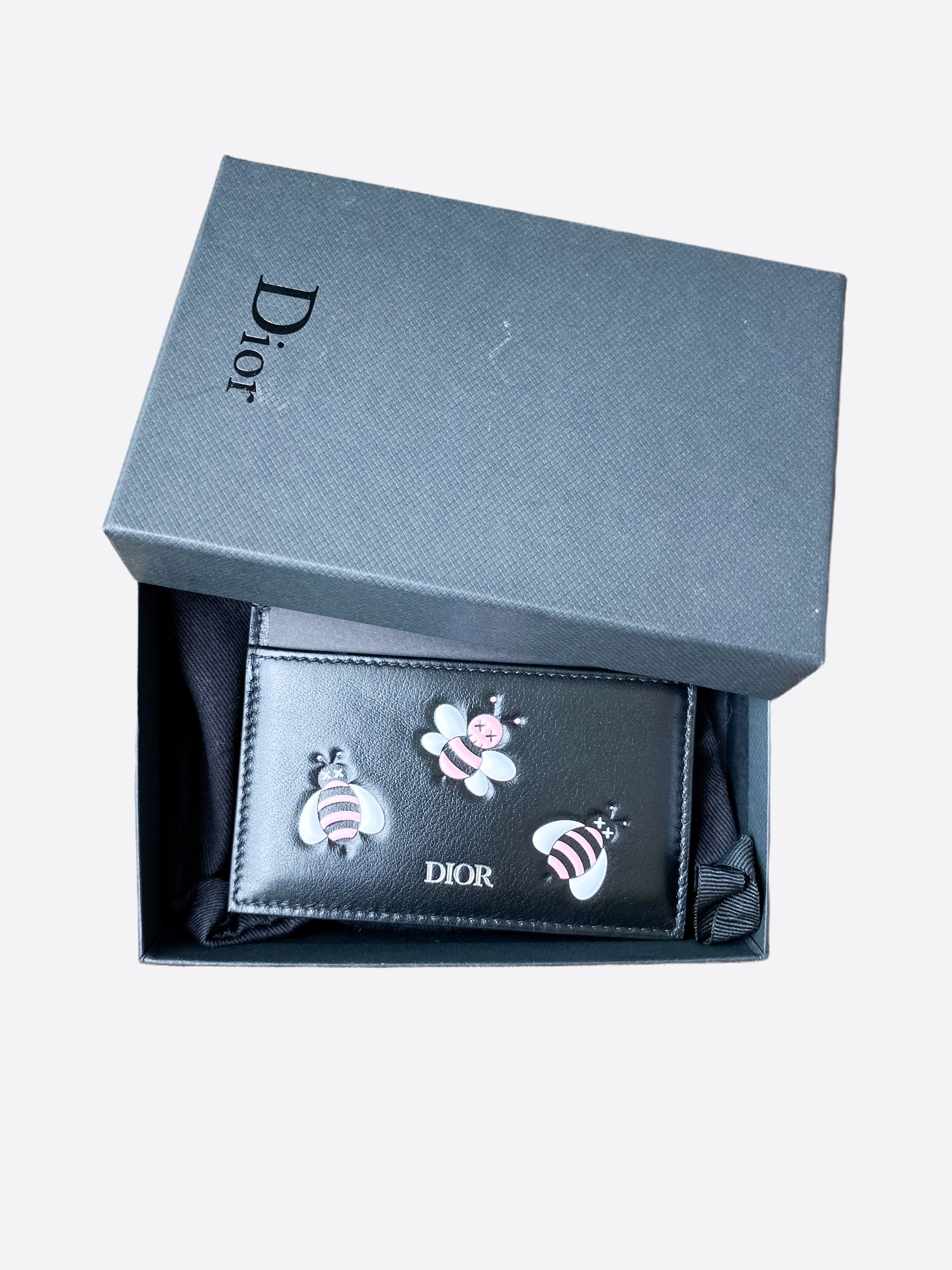The image shows a Dior jewelry box, dark gray or steel-colored, with a textured surface and "Dior" printed in gold letters on the lid. The lid is open, resting partially on the box, revealing the interior lined with black fabric. Inside lies a black leather wallet, which could either be a bifold or a card holder. The wallet has "Dior" embossed in gold on the front. Adorning the wallet are three distinct bumblebee decals, each with different styles. Two bees have single wings while the third has double wings; all are yellow and black with white wings and X-shaped eyes. The bees are positioned in varied directions, enhancing the whimsical design of the wallet.